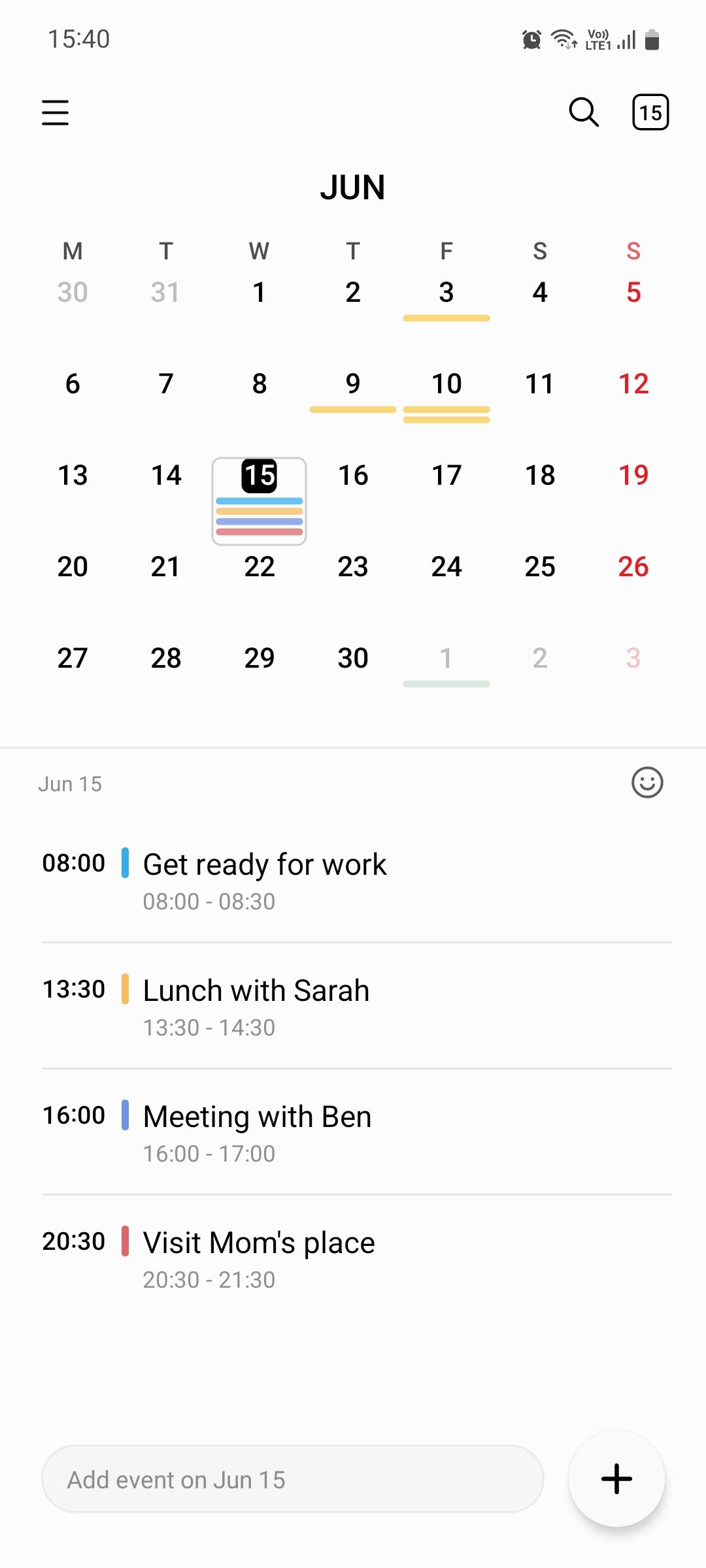This is a detailed screenshot of a smartphone's calendar app interface. At the top, there's a timestamp displaying 15:40, along with several icons indicating connectivity and battery status: a clock, Wi-Fi icon, LTE symbol labeled "LTE1 VOJ," and a battery icon showing approximately 50% charge.

Below the status bar, there is a hamburger menu icon on the left, followed by a search bar, and the number "15" displayed in a box. The calendar is set to the month of June, with the 3rd, 9th, and 10th dates underlined. The 10th is emphasized with a double yellow underline. The current date is the 15th, which is highlighted with a box around it.

The events for June 15th are listed vertically as follows:
- **June 15th, 08:00** - "Get ready for work" with a smiley face icon to the right. (08:00 - 08:30)
- **June 15th, 13:30** - "Lunch with Sarah" (13:30 - 14:30)
- **June 15th, 16:00** - "Meeting with Ben" (16:00 - 17:00)
- **June 15th, 20:30** - "Visit mom's place" (20:30 - 21:30)

At the bottom, there is an option to add a new event for June 15th, indicated by a "plus" button symbol.